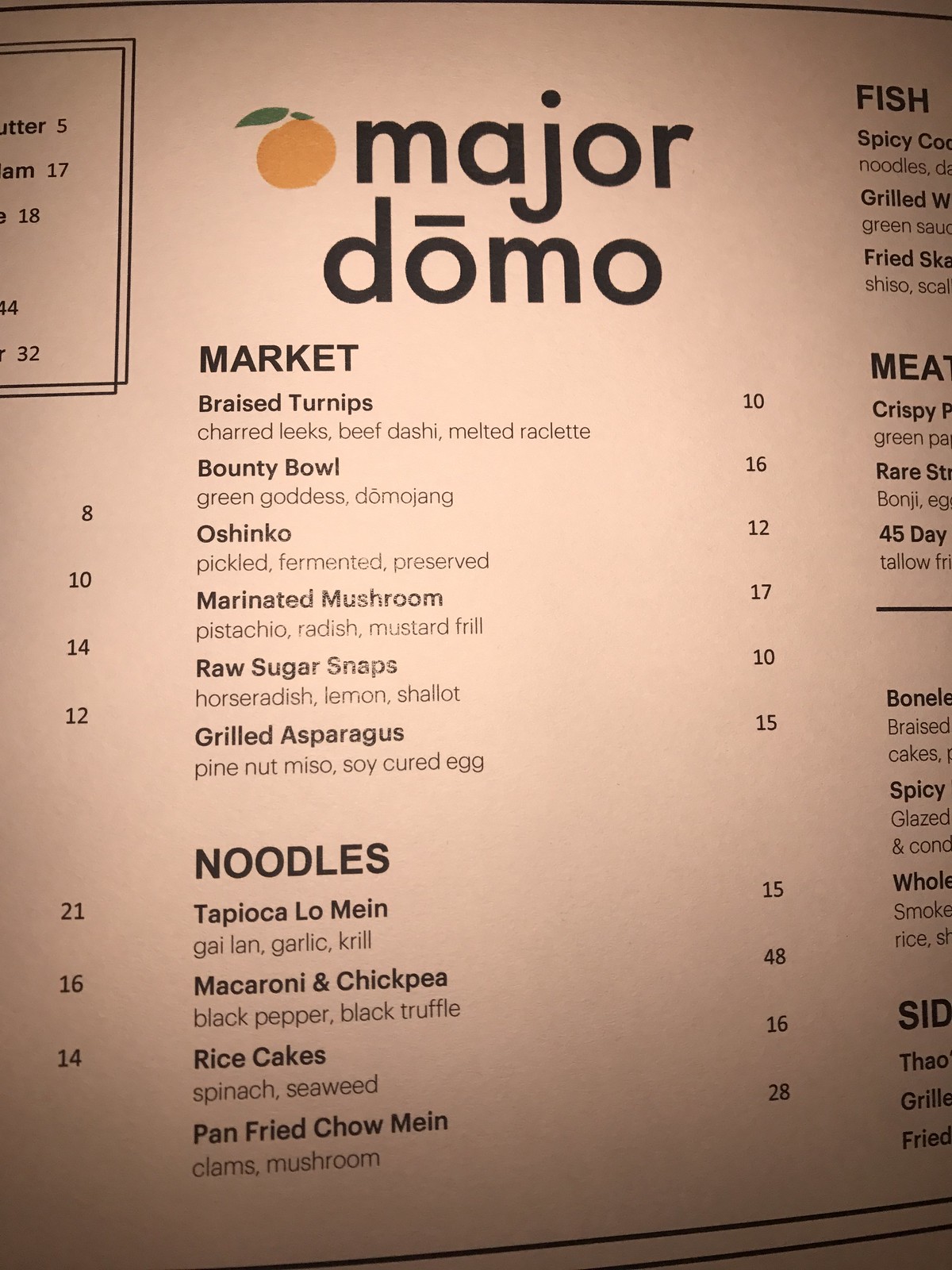The menu page is elegantly presented with black text printed on light amber-tinged paper, offering a warm and inviting aesthetic. Various menu items are listed under the market segment, showcasing a range of sophisticated dishes. These include Braised Turnips priced at $10, a Bounty Bowl for $16, Oshinko for $12, and Marinated Mushrooms for $17. Further options include Raw Sugar Snaps at $10, Grilled Asparagus for $15, Noodles and Tapioca Lo Mein each listed at $16, Macaroni and Chickpea for $48, Rice Cakes for $16, and Pan Fried Chow Mein priced at $28. Moving to the right side of the image, the menu extends to feature sections on fish, meat, and sides, though the complete details of these items are not fully visible. The carefully curated selection and the traditional yet sophisticated print design suggest a refined dining experience.